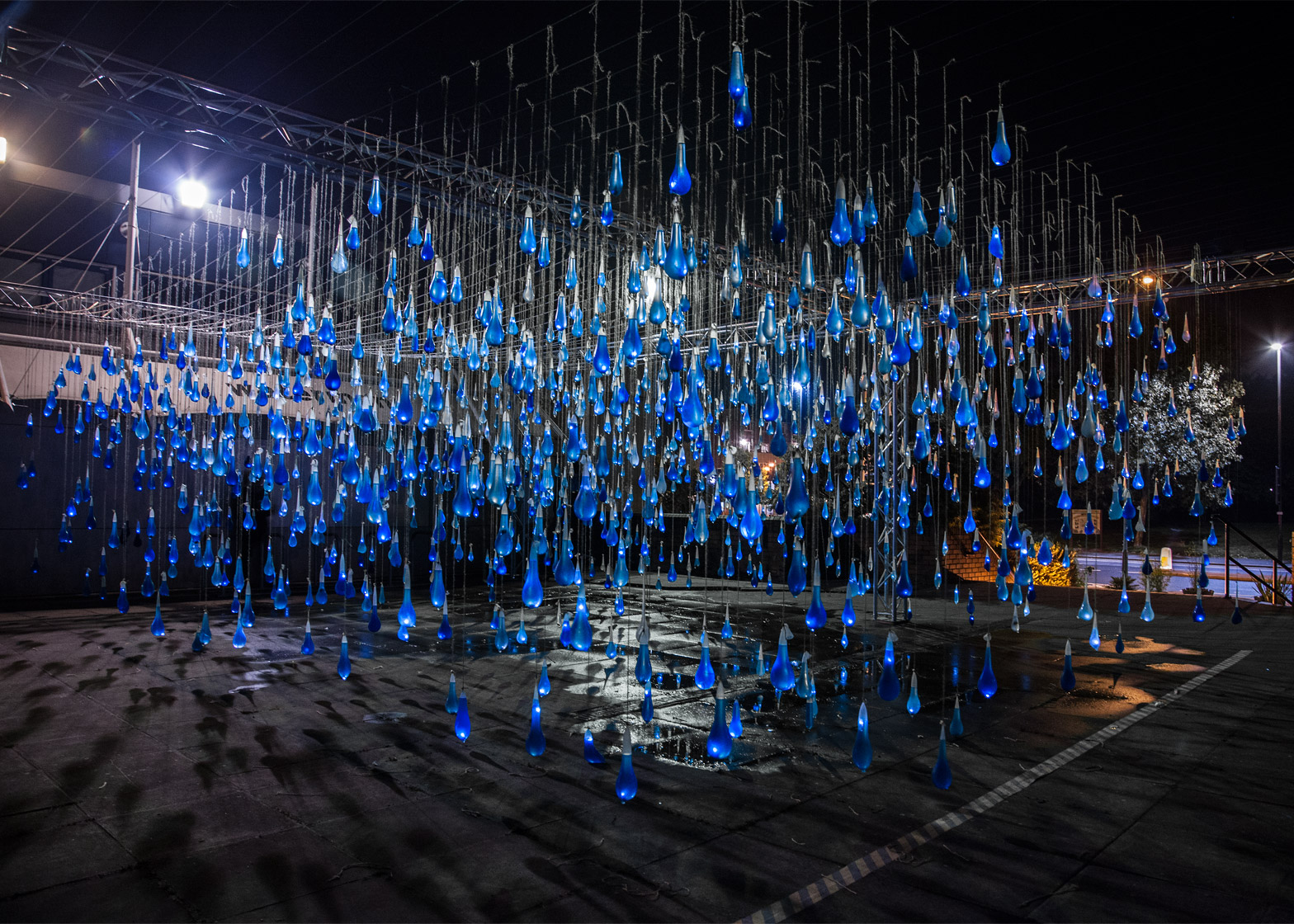The image appears to be a nighttime outdoor art installation, evocative of rainfall. The scene features a black ground, possibly resembling an asphalt surface or a tarp, reflecting light in various places, mimicking the effect of wetness from recent rain. Dominating the upper portion of the image, a wire framework suspended from above forms a crisscross pattern with wires spaced just a few inches apart. From these wires, hundreds of translucent royal blue vials dangle at varying lengths, creating an illusion of raindrops or teardrops falling from the sky. These vials, which resemble upside-down light bulbs, are uniformly three to four inches long and a couple of inches wide, allowing light to shine through them and enhancing their resemblance to falling water droplets.

The installation's dark ambiance is pierced by a few light sources: a prominent light post stands to the left behind a metal fence, and another distant light adds to the whimsical illumination. To the right, there seems to be part of a bench and more fencing visible, reinforcing the setting in a possibly recreational outdoor area like a tennis or basketball court. The combination of suspended blue vials and reflective surfaces effectively simulates a vivid scene of rain, with the entire setup creating a surreal, mesmerizing representation of rainfall at night.